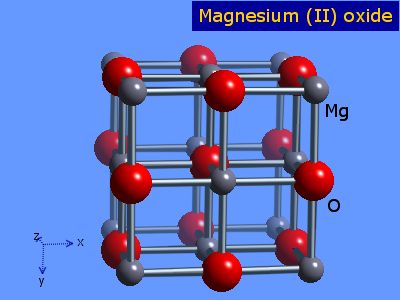This is a detailed diagram depicting the atomic structure of magnesium oxide. The entire image is set against a light blue background. In the top right corner, a dark blue square with gold lettering spells "magnesium oxide," with the chemical symbols: a capital "M" followed by a lowercase "g" (Mg) and a lowercase "o" (O). The diagram features a repeating structure across three levels, arranged in a three-by-three grid, each with distinct yet mirrored properties.

At the front plane, a silver square grid hosts spheres, with a vertical and horizontal central line segment dividing it. The central part is occupied by a big red ball (representing oxide, O) at the north, south, east, and west locations around the vertical and horizontal midlines. These are interconnected by smaller gray balls (representing magnesium, Mg) at each corner of the square and at the intersection points across both lines.

The middle plane mirrors the front but with the positions of the red and gray spheres swapped: larger red balls take the place of the previous gray ones and vice versa.

The back plane replicates the arrangement of the front layer, maintaining the same color spheres in their respective positions.

The small gray spheres, labeled with "Mg," represent magnesium atoms, while the red spheres marked with an "O" symbolize oxide ions. The layout of these spheres in a grid-like formation elaborately conveys the layered structure of magnesium oxide. The entire diagram, detailed with color-coded spheres and precise annotations, enhances our understanding of this compound, resembling a visual aid from a science textbook.